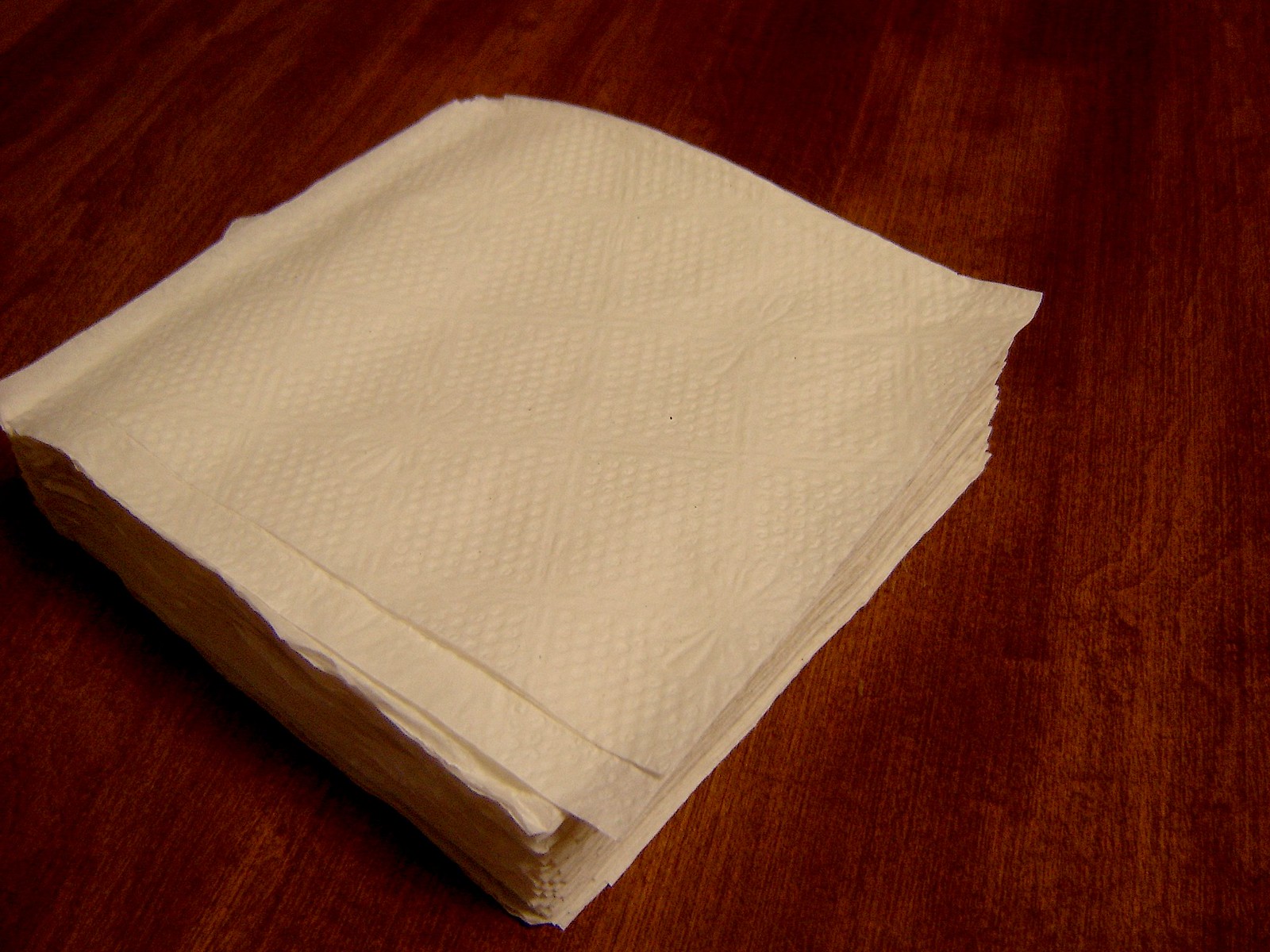This horizontal, rectangular color photograph depicts a neatly stacked pile of approximately 25 to 30 plain white paper dinner napkins, set on a dark reddish-brown wood grain tabletop, possibly cherry or walnut. The white napkins are square in shape and feature a delicate, slightly dimpled texture with an embossed flower pattern. The napkins are primarily stacked directly on top of one another, except for the topmost napkin, which is slightly askew and overhangs the stack. The arrangement of the napkins forms a diamond shape, and the stack is positioned closer to the left side of the image, with the left edge of the pile partially cut off. The lighting is somewhat dim, casting a subtle shadow beneath the napkins on the left side, highlighting the table's polished surface.